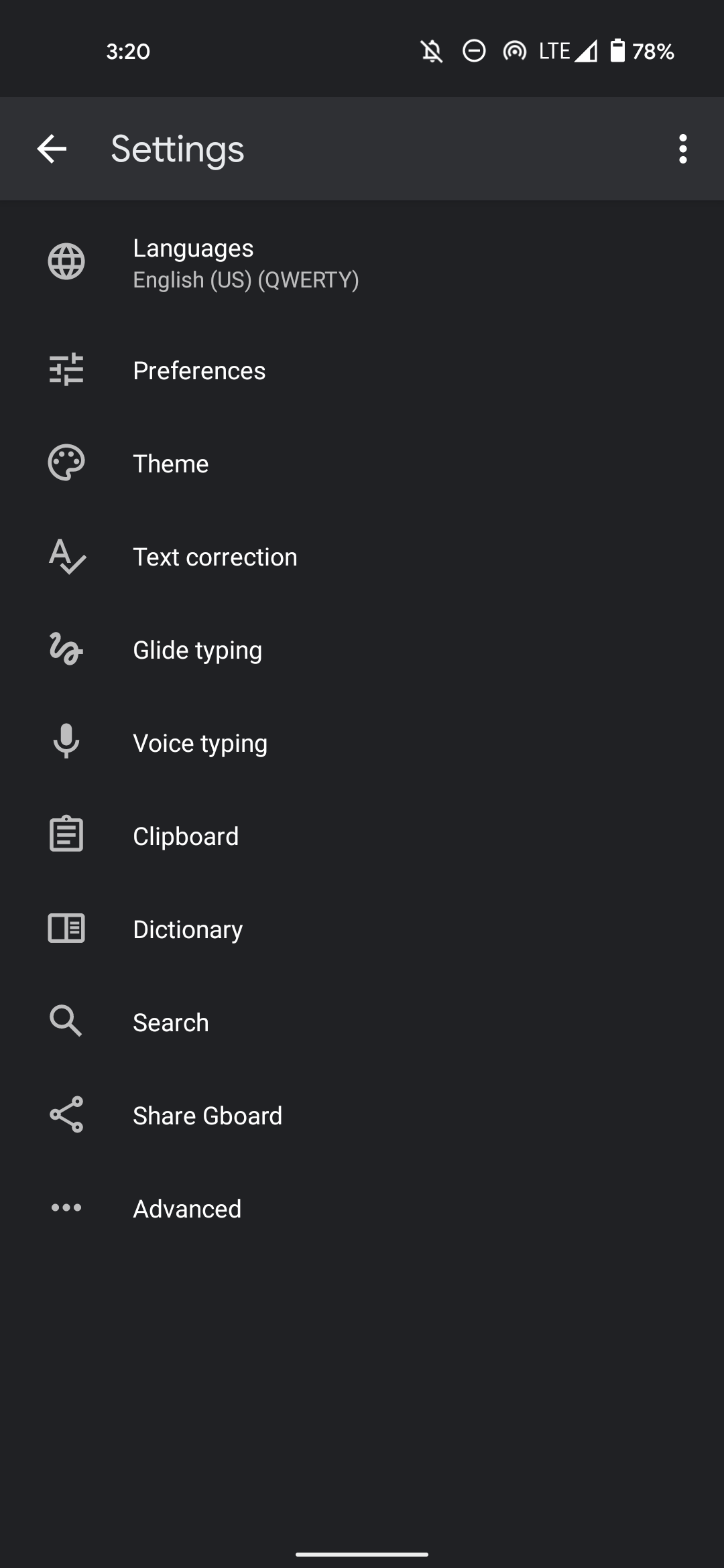The image displays a smartphone settings menu against a black background, with all text and icons in white for high contrast. At the top of the screen, there is the status bar showing a muted bell icon, the number "320," a circle and line icon, an "LTE" signal indicator, and a battery icon.

Heading down the screen, the first line reads "Settings," accompanied by a back arrow and three vertical dots indicating additional options. Below this, the menu begins with several settings categories:

1. **Languages** - Represented by a globe icon. It specifies "English, U.S., QWERTY" layout.
2. **Preferences** - Indented with line icons.
3. **Themes** - Illustrated by an artist's palette with paint.
4. **Text correction** - Denoted by an "A" with a check mark.
5. **Glide typing** - Symbolized by a squiggly line.
6. **Voice typing** - Marked with a microphone icon.
7. **Clipboard** - Shown with a clipboard icon.
8. **Dictionary** - Represented by an open book icon.
9. **Search** - Depicted with a magnifying glass icon.
10. **Shared** - Refers to "Gboard" and is displayed with a triangular icon.
11. **Advanced** - Highlighted with three white dots.

At the bottom of the screen, there's a white bar, but no additional information or notable visual elements are present. The image showcases a clear and user-friendly display, likely a sub-menu from a smartphone's settings screen. The design appears straightforward and easy to navigate.